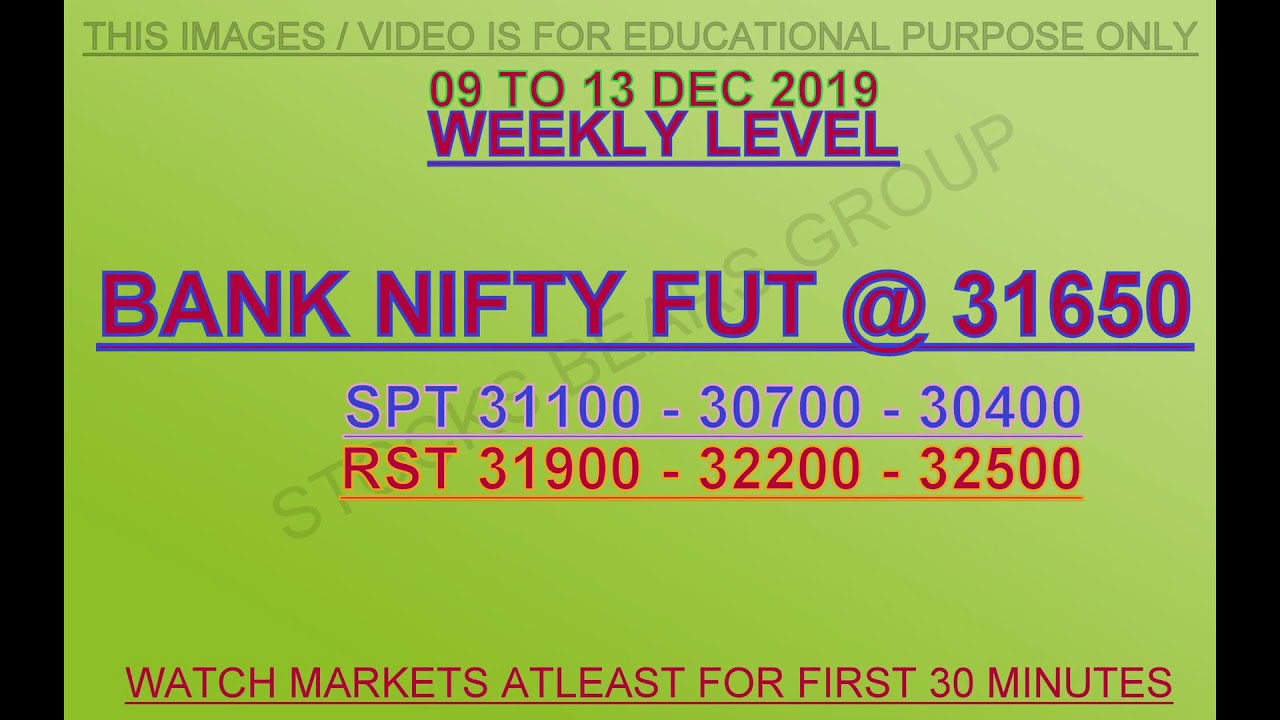The image depicts an announcement on a gradient light green background, with green gradients that are lighter at the top right-hand corner and darker at the bottom left-hand corner. Centered at the top, in white text, are the words: "This image/video is for educational purpose only," underlined with a light gray line stretching across the width. Below it, in bold red text, it states "09 to 13 DEC 2019," also underlined. Centrally positioned on the green background, in large purple text with a blue outline, is the title "Weekly Level," underlined with a blue line. Further down, highlighted in bold purple text with a blue outline, it reads "Bank Nifty FUT at 31650." Underneath, in blue text, it lists "SPT 31100-30700-30400," underlined with a light purple line. Below this, in striking red text, it shows "RST 31900-32200-32500," followed by a red line. Finally, at the bottom, in red text, it advises, "Watch markets at least for first 30 minutes," underlined with a line of the same color.